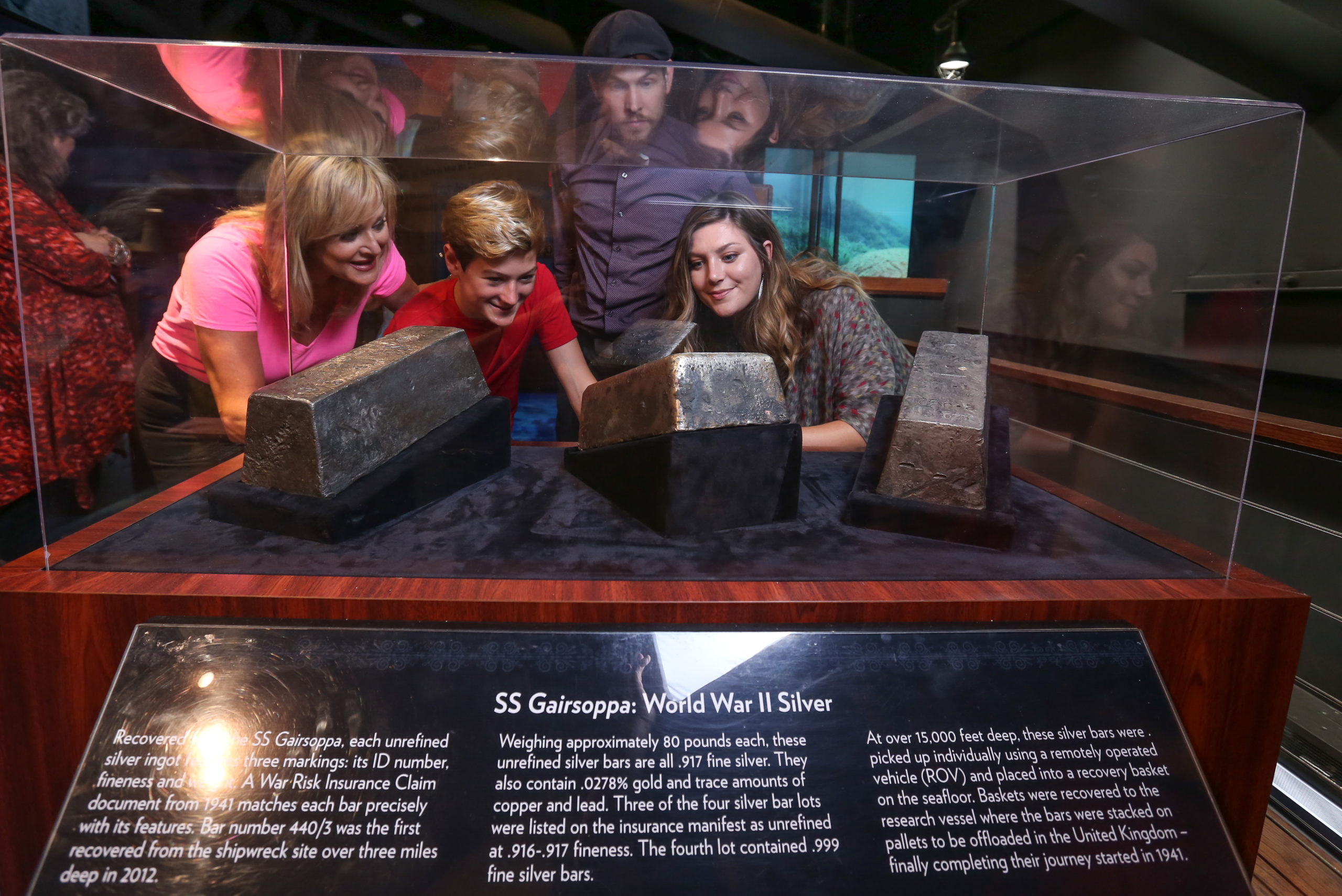A family of four is intently viewing a museum exhibit behind glass, featuring large unrefined silver bars recovered from the SS Gairsapa, a World War II ship. The silver, weighing approximately 80 pounds each and marked as .917 fine with traces of gold, copper, and lead, are displayed atop a black cushioned surface within a wooden structure. The text on the display, partially obscured by glare from overhead lights, details that three of the four lots listed on the insurance manifest were .916 to .917 fineness, with the fourth being .999 fine silver. The family includes a boy in a red t-shirt and dirty blonde hair, a girl in a gray top also with dirty blonde hair, a bearded man in a purple shirt, and a woman in a pink top with black slacks. Behind them, the reflections in the glass hint at more spectators and a nearby aquarium setup seen through a window, all framed by wooden floors. Everyone is smiling, absorbed by the historical treasures before them.